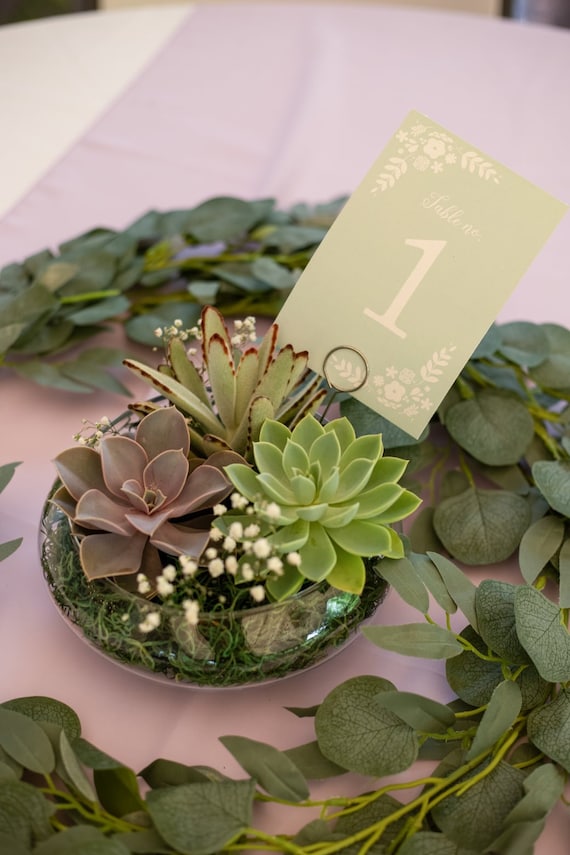The image depicts an elegantly set round table covered with a white tablecloth, viewed from overhead. At the center of the table is a clear, circular glass planter bowl filled with an arrangement of artificial succulents. Green succulents are positioned on the right side, while purplish ones are on the left, accompanied by a lighter green succulent towards the back. The planter is accented with small white flowers and faux green grass. Surrounding the planter is a wreath-like arrangement of lime green eucalyptus stems, each adorned with bunches of oval-shaped leaves, forming a circular pattern around the bowl. In the center of this setup, a light olive-green card with "Table 1" printed on it is held by a small holder, indicating the table number for the event. The overall centerpiece combines various textures and hues, creating a visually appealing and cohesive decoration.